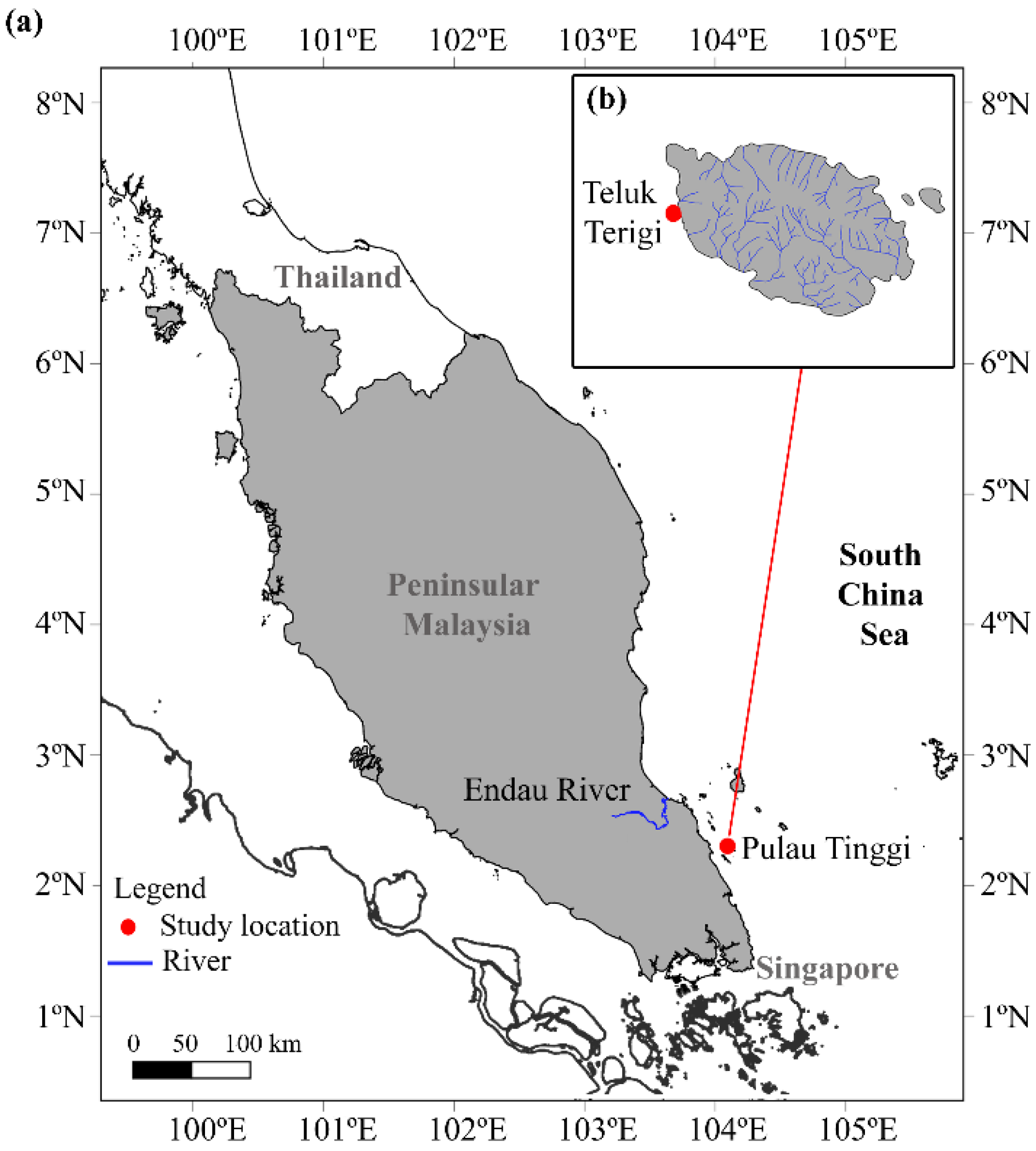This detailed map displays the geographic region encompassing Thailand and Peninsular Malaysia, featuring prominent natural landmarks and coordinates. The map is primarily black, white, and gray, with blue and red highlights for specific elements. Central to the map is a large landmass labeled Thailand, which includes the Endau River, Peninsular Malaysia, Pulau Tinggi, and Singapore. To the east, the South China Sea is marked. 

An inset in the upper right corner shows a smaller map of Pulau Tinggi, denoted as a study location. The map's legend explains the symbols used: a dot signifies study locations, blue lines represent rivers, and the red is used to highlight the Endau River. Longitude lines run from 100 degrees east to 105 degrees east along the bottom and top, while latitude lines from 1 degree north to 8 degrees north span both the left and right sides of the map. This thorough depiction provides a comprehensive view of the region's geography, including key landforms and water bodies.